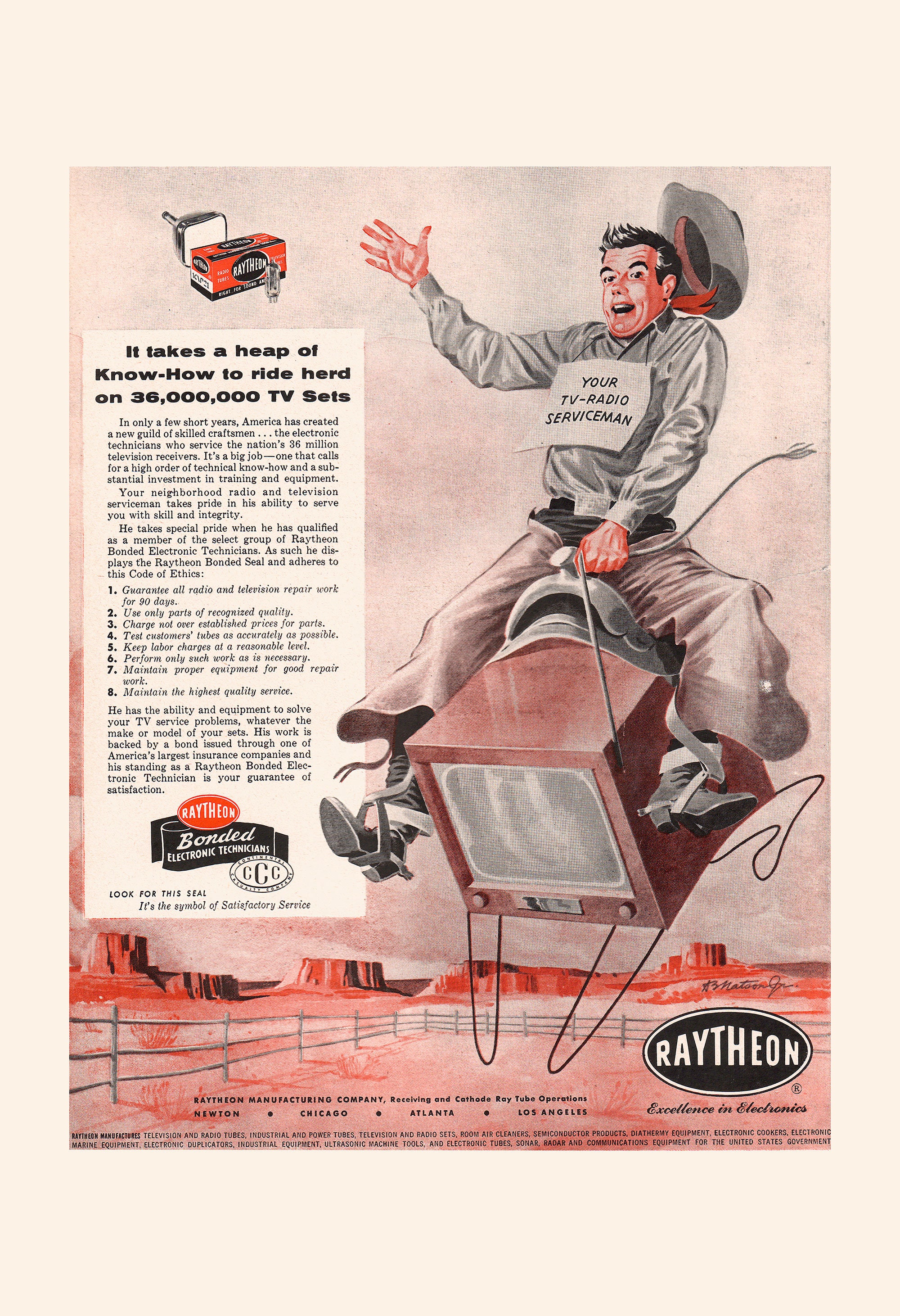This 1950s-style hand-drawn advertisement for Raytheon Corporation features a vivid and playful illustration of a TV service repairman dressed as a cowboy. The central image depicts the repairman in a silver uniform with a bib reading, "Your TV Radio Serviceman," as he rides a bucking television set equipped with a saddle and stirrups, akin to a wild horse or bull. His hat is flying off, adding to the dynamic and whimsical scene. A cathode ray depiction of an old television set, accompanied by a box displaying the Raytheon logo, occupies the upper portion of the ad. On the left side, there's a column of text, though mostly too small to read, with the prominent headline stating, "It takes a heap of know-how to ride herd on three million TV sets." The advertisement predominantly features reds, oranges, browns, and grays, enhancing its vintage appeal. At the bottom right corner, the classic Raytheon logo is prominently displayed within an oval. The backdrop is a pinkish hue, further cementing the nostalgic 1950s aesthetic.